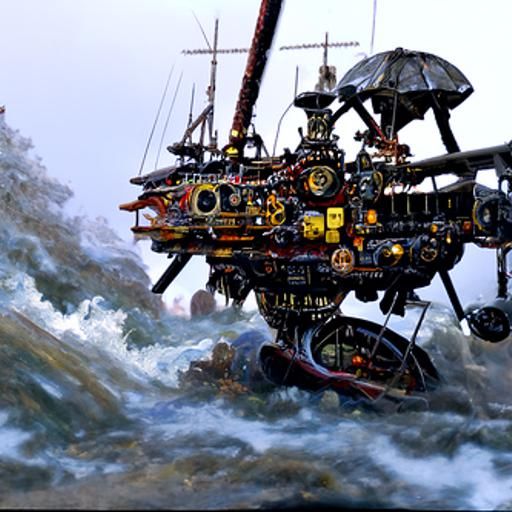The image appears to be an animated or digitally created depiction of a wildly imaginative ship navigating through turbulent waters. Dominating the right side of the scene, the vessel is a blend of fantastical elements and vibrant colors. The hull is an intricate patchwork of red, yellow, blue, and black geometric shapes, featuring multiple circular and rectangular panels that lend it an almost robotic appearance. A large, imposing mast rises near the front of the ship, slightly tilting and continuing off the top edge of the image. Accompanying the mast are light-colored cross-like structures that add to the ship’s unconventional design. Toward the rear, the ship sports an umbrella-like apparatus and a peculiar structure resembling a seat, beneath which a row of bead-like forms can be seen. It also has large, porthole-like circles, and a long plank seems to stretch out beyond the image's right edge. The vessel’s base has a rounded form akin to a submarine, merging into a broad, open rudder or stand. Surrounding the ship, the scene is filled with dynamic water elements: large, crashing waves on the left, some gray waves to the right, and a rocky outcrop protruding from the bottom, enveloped in frothy white water. This tumultuous seascape enhances the adventurous and otherworldly aura of the ship.